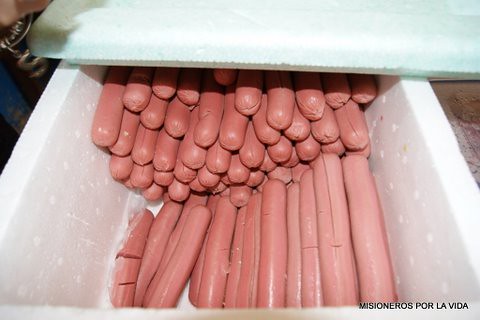The image is a color photograph of a large number of raw hot dogs stacked in a pyramid-like formation inside a white styrofoam cooler. The cooler, which occupies most of the frame, has its lid removed and positioned sideways to reveal the contents, casting a shadow on the edge. At the bottom right of the image, small black print reads "Misioneros por la Vida," indicating a possible connection to a humanitarian mission. The scene has a somewhat unappetizing appearance, primarily dominated by the pale hue of the hot dogs and the stark white of the cooler. A barely visible human hand appears in the upper left corner, adding a hint of additional context to the setup. Overall, the image conveys a preparation scene likely intended for a charitable purpose.